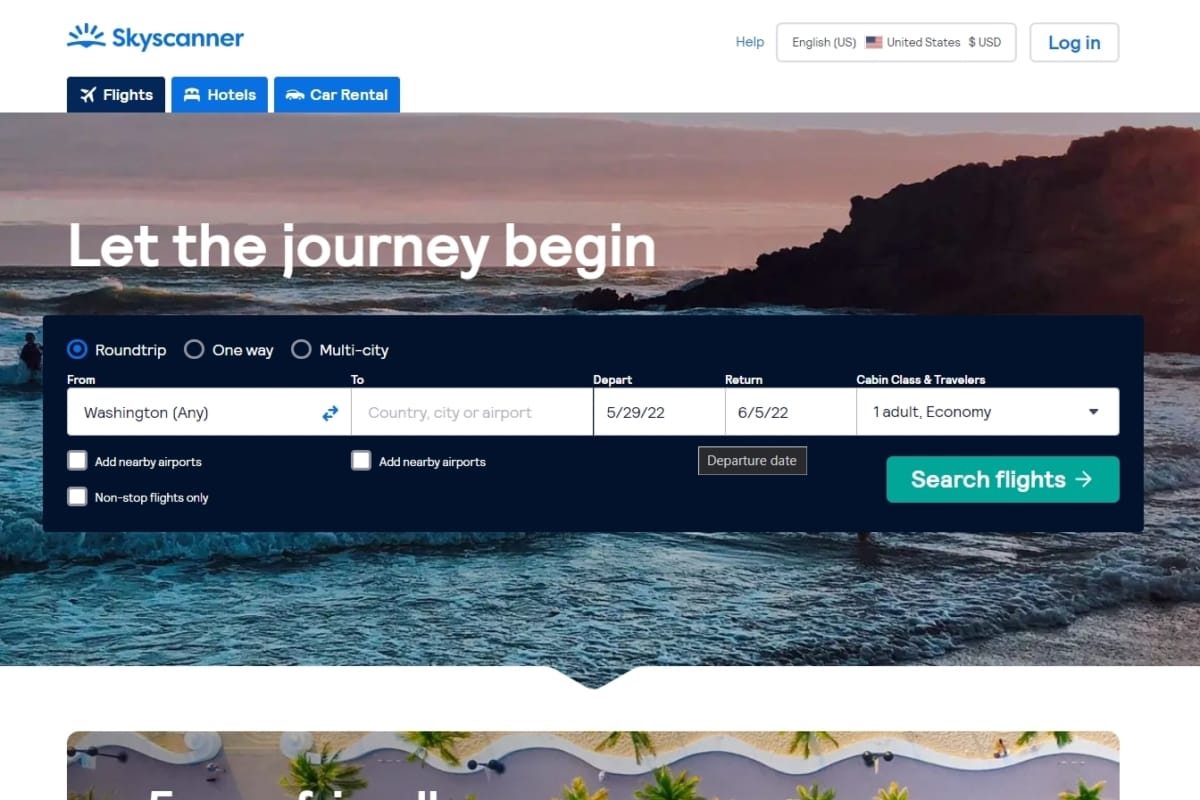Screenshot of the Skyscanner Website

In this screenshot, the Skyscanner website is prominently displayed. The top left corner features the Skyscanner logo, which depicts an airplane with a sun rising behind it. On the top right, there are links labeled "Help," "English (United States)," and "USD - United States Dollar," along with an option to "Log in."

Beneath the Skyscanner logo, navigation tabs for various services are clearly visible, including options for "Flights," "Hotels," and "Car Rentals." Dominating the central part of the page is a rectangular banner image that shows a scenic view of the sky with a rock formation jutting into the ocean. Superimposed over this picturesque background is a motivational message: "Let the journey begin."

Just below this banner, options for booking flights are arranged. Users can select between "Round-trip," "One-way," and "Multi-city" flights. The journey is preliminarily set from "Washington" to an unspecified destination. Travel dates are from May 29, 2022, to June 5, 2022, and the trip is intended for "one adult" traveling in "economy" class.

Additional search preferences are represented by a series of unchecked boxes, which include options to "Add nearby airports," search for "Non-stop flights only," and select a "Departure date." Finally, a prominent "Search flights" button with a right-pointing arrow invites users to commence their flight search.

This comprehensive layout and clean design aim to facilitate an effortless and efficient flight booking experience.